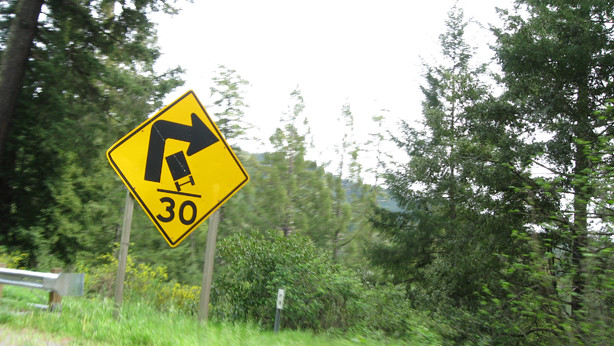In the photograph taken outside, a heavy overcast white sky looms over a scenic roadside view. In the distance, a hill covered with trees can be seen, while closer to the camera, a row of pine trees with bushes at their bases lines the scene. Towards the foreground, a slight incline leads up to a metal guardrail, beside which stands a small white sign. Prominently in front of the guardrail, two pieces of wood jut out from the ground to support a yellow diamond-shaped road sign. The sign features a black border and a right-turning black arrow, alongside an image depicting a car tilting, indicative of a sharp turn. Below this graphic, the number '30' is clearly displayed. The area is lush with greenery, creating a contrast with the structured elements of the road signage and guardrail, capturing the tranquil yet orderly intersection of nature and infrastructure.